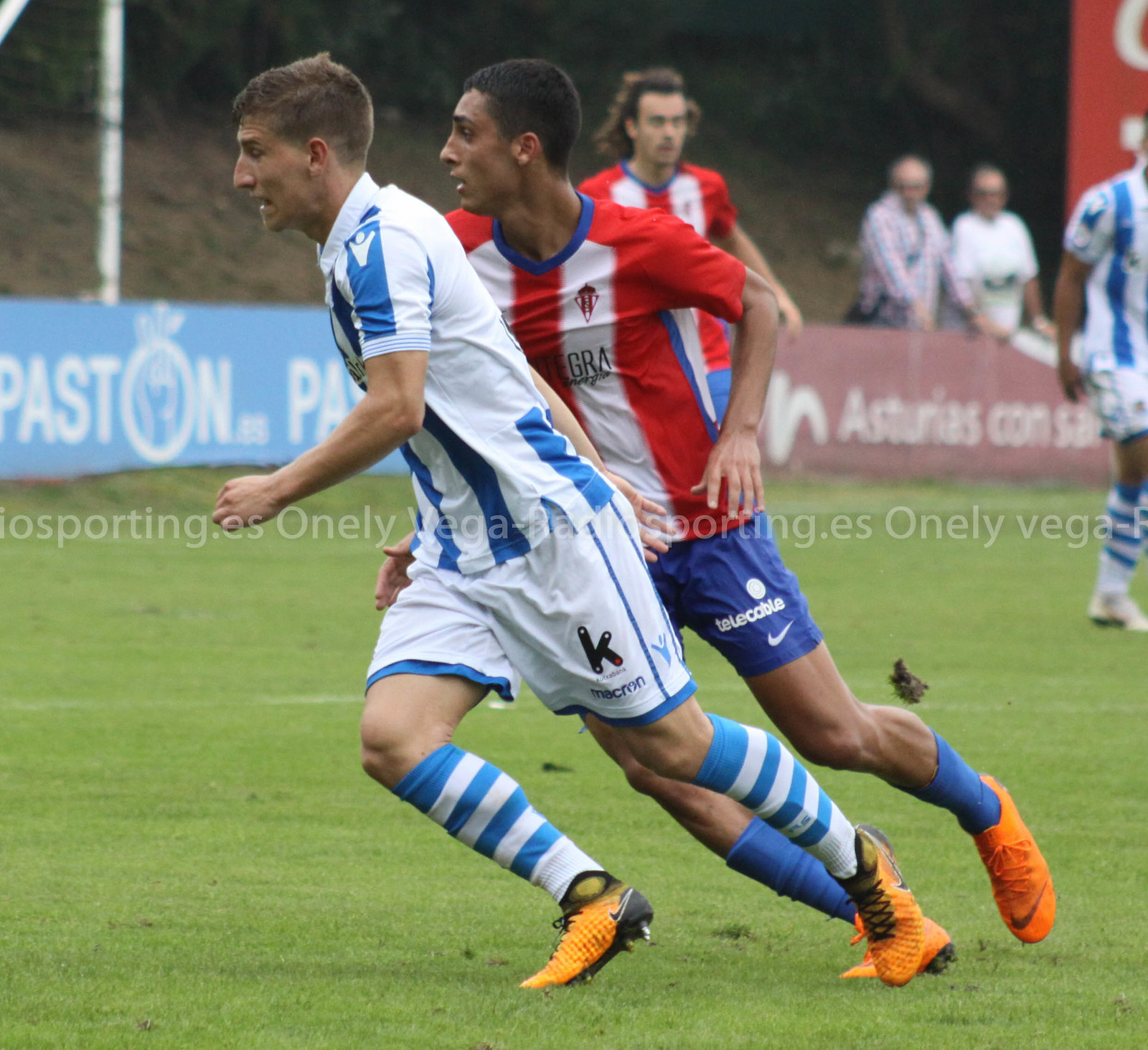In this dynamic action shot from a soccer game, two players sprint side-by-side, their focus intensely on the unseen ball. The player on the left wears a white and blue uniform, complemented by matching striped socks and vibrant orange and black cleats. His counterpart, donned in a red and white vertically striped jersey with a blue collar, sports blue shorts, blue socks, and orange cleats as well. Behind them, the field's edges are lined with advertisements for companies like "Paston" and "Asturias" and a watermark reading "onelivega.somethingsporting.es" is faintly visible. Sparse spectators, including a discernible photographer, watch the unfolding action. In the background, a few teammates stand by, attentively following the run of these two players.